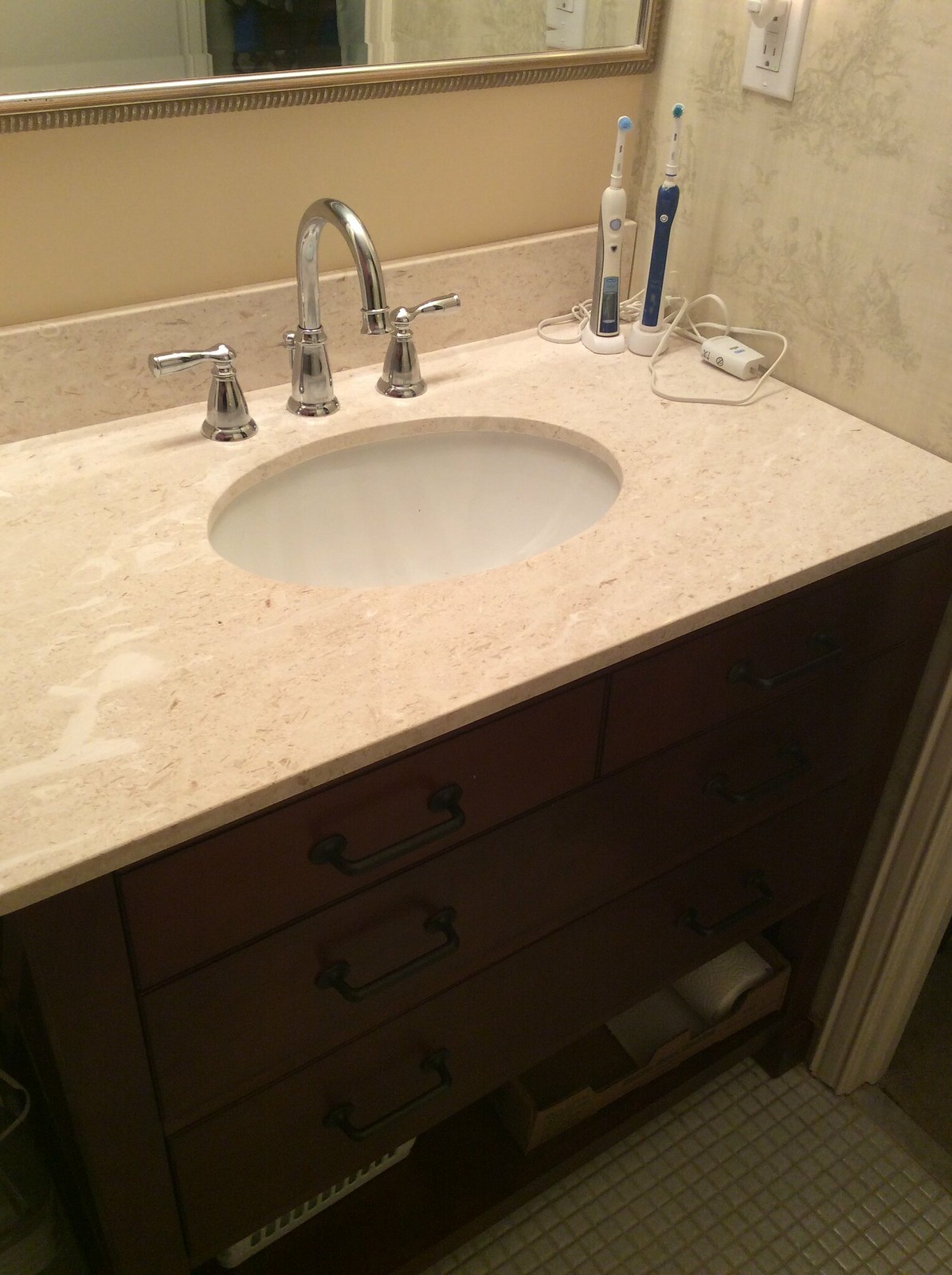In the image, we see a bathroom sink set atop a luxurious marble countertop with an oval cutout. The pristine white sink is complemented by sleek silver fixtures. This ensemble is mounted on a rich, dark brown wooden cabinet featuring three drawers adorned with black handles. Beneath these drawers lies an open shelf area that houses a white basket, partially obscured by an unidentified object.

The floor is tiled with small, penny-sized, light to medium brown tiles that have been grouted in a matching brown. To the right of the sink, two electric toothbrushes are positioned with their cords coiled in a heap, though not plugged into the nearby white electrical outlet. This outlet is embedded in the same elegant marble that tops the sink area.

Above the sink, a mirror framed in gold adds a touch of opulence. The wall behind the mirror is painted a light tan, seamlessly blending with the overall aesthetic of the bathroom. The surrounding decor ties together elements of elegance and functionality, captured in remarkable detail.